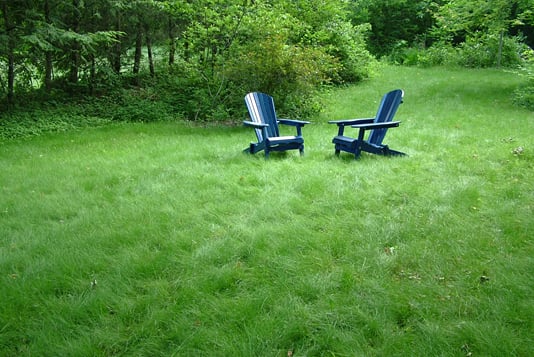The photograph captures a lush, green outdoor scene, likely a tranquil backyard, where the dominant feature is the vibrant grass, appearing unmowed for about two weeks and covering the majority of the lower half of the image. At the center, slightly down from the top edge, are two beautifully crafted Adirondack chairs made of wood, painted in a striking, shiny navy blue. The chairs are positioned facing each other, inviting a comfortable conversation. Behind them, there's a small clearing continuing the expanse of verdant grass. Surrounding the scene, trees in varying shades of green frame the left-hand side and extend from the top right to the top left corners of the image, adding depth and a natural enclosure. Additionally, directly behind the chairs, a lush, un-groomed green bush adds to the vibrant, untamed feel of the setting. The presence of sunlight suggests that the photo was taken during the daytime, emphasizing the luxuriant and inviting ambiance of this green haven.